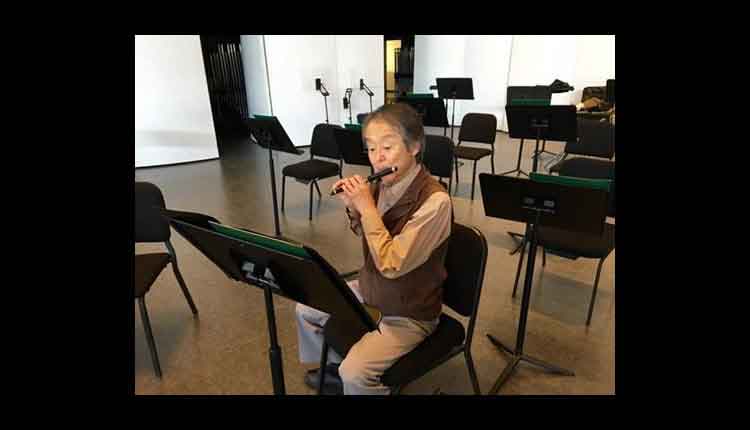The image depicts an elderly Asian woman seated in a music practice room, playing a piccolo, a shorter version of a flute. She is dressed in a brown vest over a lighter brown collared shirt, with brown pants. She sits in a black chair, amidst several rows of similar chairs and black music stands, each with a long black rod and backrest, scattered throughout the room. The light brown floor contrasts with the white back wall, which features two open doors. The photograph is slightly blurry and framed by black borders, giving it a letterboxed appearance. The woman is focused on her sheet music while holding the piccolo with her right hand from the bottom and her left hand bent at the elbow, back of the hand facing the camera.